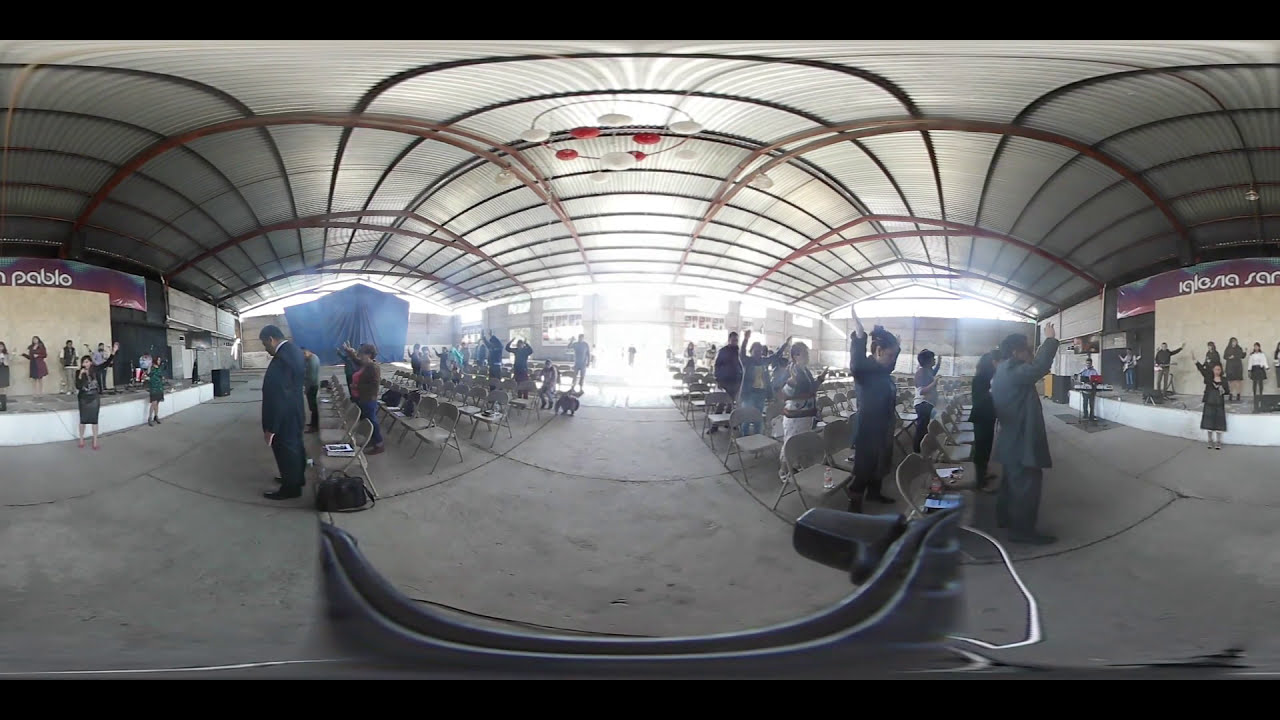In the image, we observe the interior of an enclosed meeting area, likely a church or a music venue, with a cement floor and metal folding chairs arranged in rows. The room is filled with people standing upright, many with their heads bowed and hands raised, seemingly amidst a worship ceremony or concert. A stage is positioned at the front, and on it, alongside several musicians holding instruments, a prominent woman stands in front of a microphone, her hand raised in the air.

The convex nature of the image provides a panoramic view, capturing mirror images of the band on both the left and right sides. Adding to the sense of symmetry, behind the stage on either side, partially visible text reads "I-G-L-A-S-I-A Iglesia" and "P-A-B-L-O." The ceiling features an open metal design with a distinctive object that has white and red circles. Bright light streams through the windows and doors at the back of the room, illuminating the scene. Scattered among the empty chairs are various personal items, such as books, left behind by those who have risen to join in the communal activity.